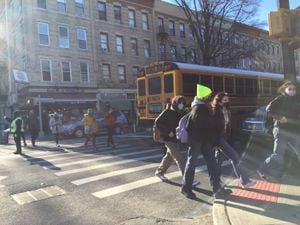The color photograph, taken during daytime, captures a bustling street intersection. The scene shows a large yellow school bus having just exited the intersection, with a group of middle to high school students, all wearing COVID masks, crossing the wide crosswalk. The sunlight, from the upper left corner, casts long shadows indicating early morning in the fall, emphasized by a leafless tree in the background. In the foreground, students with backpacks and winter clothing are about to step onto the curb. To the left, a crossing guard, dressed in black with a neon green vest, ensures their safety. Behind them lies a four-story apartment building, stretching across the frame, with cars parked in front. The overall atmosphere conveys a typical school morning in a city setting.